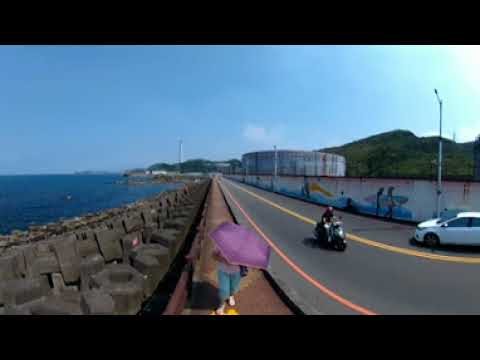A grainy, blurry daytime photograph captures a busy city street scene with a vertical, rectangular composition bordered by horizontal black stripes at the top and bottom. At the top, a bright blue sky with sunlight shining from the upper right corner illuminates the area. The street itself, featuring dark gray pavement, is marked with yellow lines on either side. A person on a black motorcycle drives down the center of the road towards the camera, while a white car moves in the opposite direction, facing left.

On the right side of the road, a gray concrete wall adorned with graffiti, which depicts scenes of people surfing, runs parallel to the street. Beyond the wall, a low, round gray building is visible, potentially a water treatment facility, with rolling green hills rising in the background.

To the left of the road, there's a series of features starting with a dark brown concrete walkway. A person, obscured by a purple umbrella and dressed in blue pants, walks along this path, heading towards the camera. Next to this walkway is a dark gray barrier, possibly rubber used for storm protection, and further left, the blue expanse of the ocean comes into view, completing the diverse and bustling cityscape.